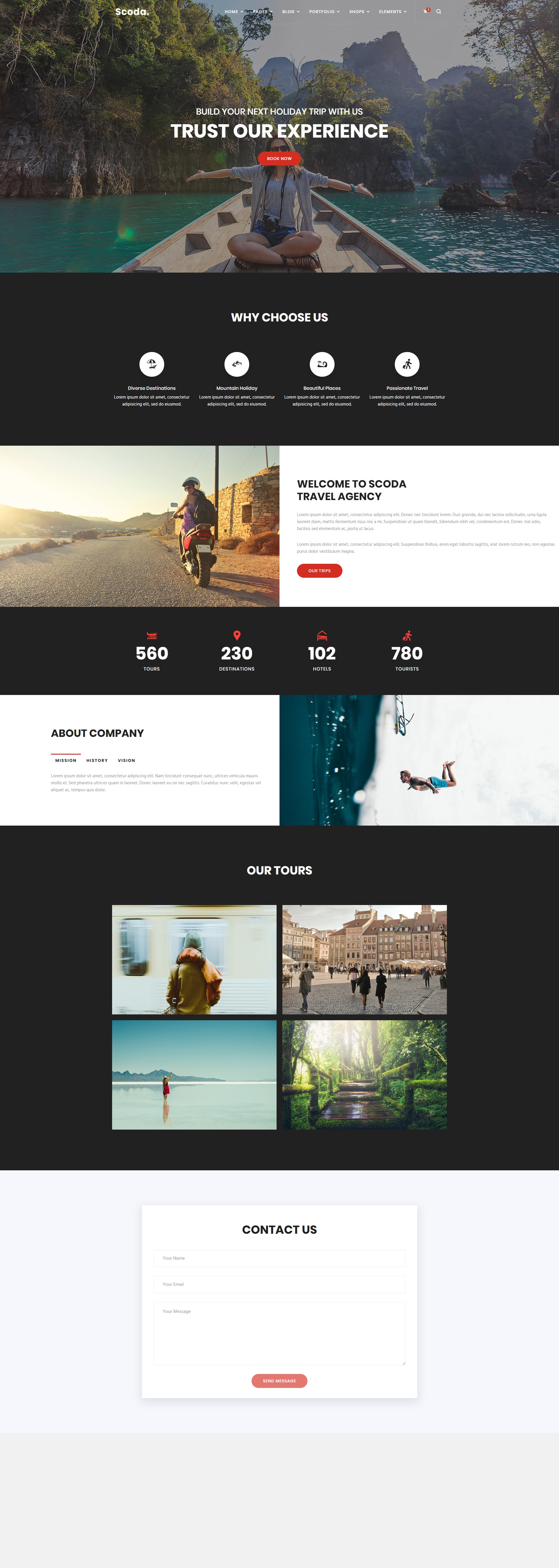**Image Caption:**

The screen capture features a highly detailed and potentially zoomed-out view of a tourist website. At the top of the screen, there is a navigation bar with various white submenu options, although the exact text is difficult to discern due to the resolution. On the top section of the webpage, there's an image of a woman sitting cross-legged on a light wood surface, dressed in a white shirt and shorts. Her arms are extended, and she is positioned next to a body of turquoise, rippling water, with a cliff face and greenery visible in the background. Above this image, a white sentence, partially readable, states “Trust our experience,” accompanied by an orange and white box.

Below this main header image, there is a black section titled "Why Choose Us." This section features four white circles, each containing a different icon, though they appear too blurry to make out distinctly. Each icon is accompanied by a brief sentence or two of white text, likely detailing key benefits or features.

Continuing down, there is another image depicting a person riding a scooter on a street. Adjacent to this image is a white box with black text, mentioning "something Travel Agency," and another orange and white box.

Further down, there's a black box displaying a series of numbers in white text paired with red icons, reading 560, 230, 102, and 780. This is likely some form of statistical or numerical information about the agency.

Following this section, a white box with two sentences of text introduces the company's details, accompanied by an image of someone in a body of water. Down the page further, there is a series of four images: one showing a person preparing to get off a subway, another of people walking in a city square, the third of an individual standing on a beach, and the last showcasing a lush rainforest.

At the bottom of the page, there is a "Contact Us" section with some text fields for user input, an orange and white submission box, and a gray box underneath it, possibly containing additional footer information or links.